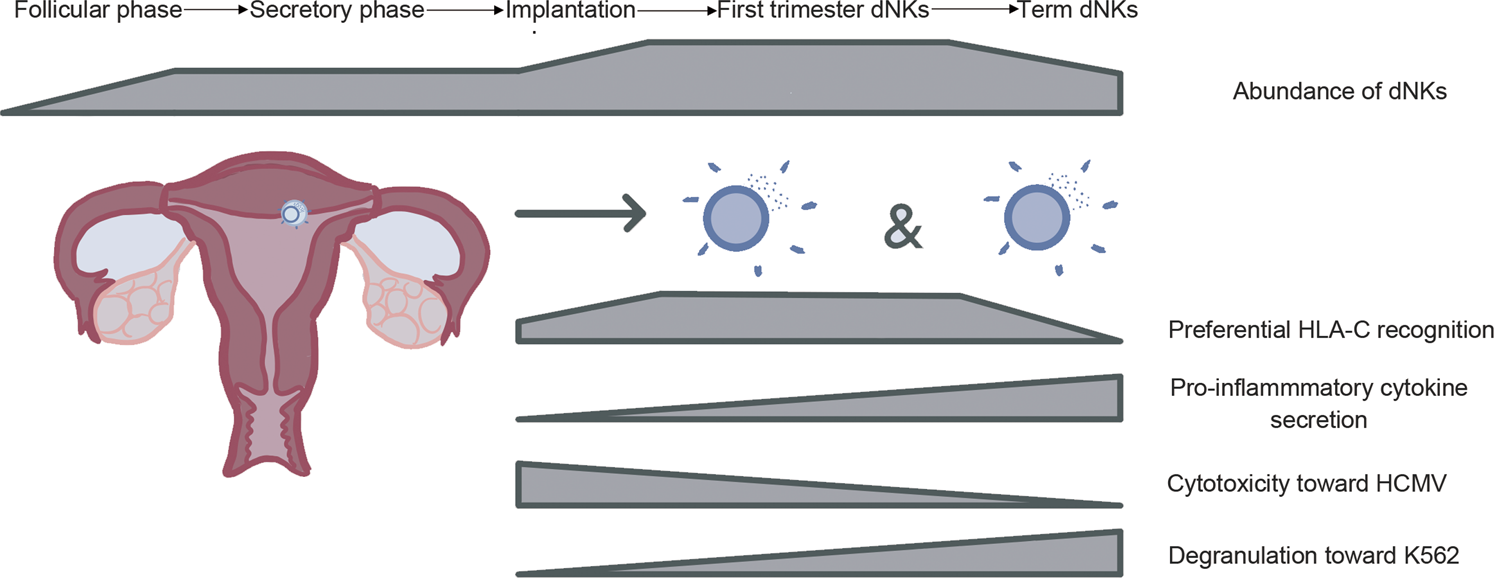The image is a detailed, scientific diagram illustrating the phases of a woman's reproductive system, specifically focusing on the menstrual cycle and associated immune responses. At the top, a timeline spans from the follicular phase to the secretory phase, then to implantation, followed by the first trimester DNKs, and finally term DNKs. 

On the left side is a detailed, colored illustration of the female reproductive anatomy, including the uterus, fallopian tubes, ovaries, and vagina. This anatomical drawing is complemented by graphical elements: an arrow points to two circular images with radiating lines, representing the egg and sperms, referred to with an ampersand between them.

The right side of the image features gray, angular shapes arranged vertically, each linked to specific medical terms and processes:
1. **Abundance of DNKs**
2. **Preferential HLA-C Recognition**
3. **Pro-inflammatory Cytokine Secretion**
4. **Cytotoxicity Toward HCMV**
5. **Degranulation Toward K562**

These descriptions highlight the immune cells' activities during the reproductive phases. The overall design, featuring detailed illustrations and specific terminology, suggests the diagram is likely educational, possibly sourced from a textbook or a scientific presentation.